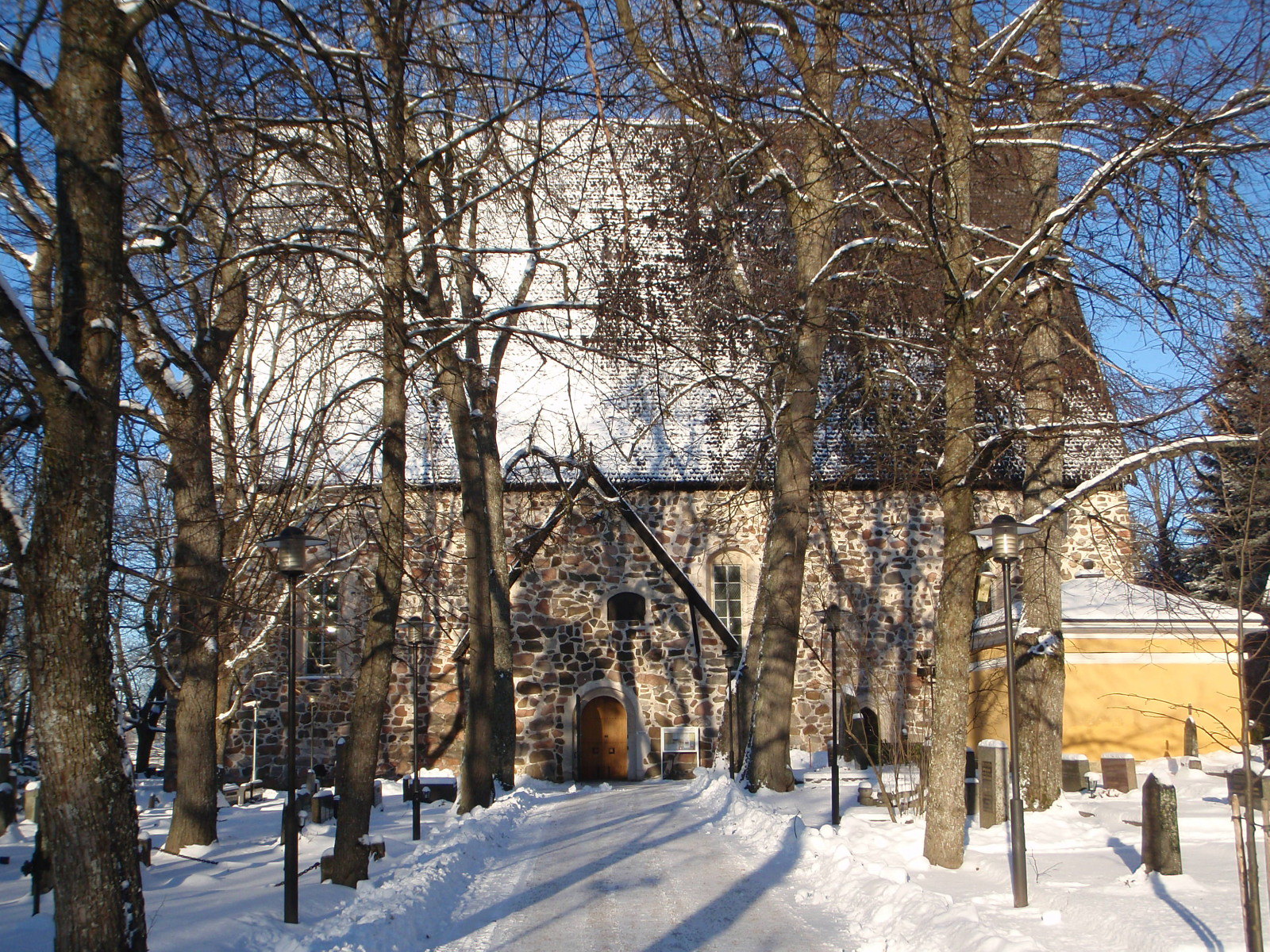In this winter scene, a large, tall stone building resembling a church stands prominently with its steeply pitched tile roof partially covered in snow. The stonework is composed of variously sized pieces meticulously mortared together, and the roof features asphalt tiles. The entrance is marked by a small arched wooden door set into a stone frame. Snow blankets the ground, but a path has been plowed leading up to the entrance.

Surrounding the building is a front yard dotted with numerous tombstones, indicating a cemetery setting. Tall, leafless trees are scattered throughout the yard, their branches also dusted with snow. Light poles line the plowed path, adding to the serene yet solemn atmosphere. To the right of the main building is a smaller yellow structure with a short roof, possibly a shed or a crematorium, further suggesting the area’s association with funerary practices. The clear, light blue sky provides a crisp backdrop to this tranquil, snow-covered scene.